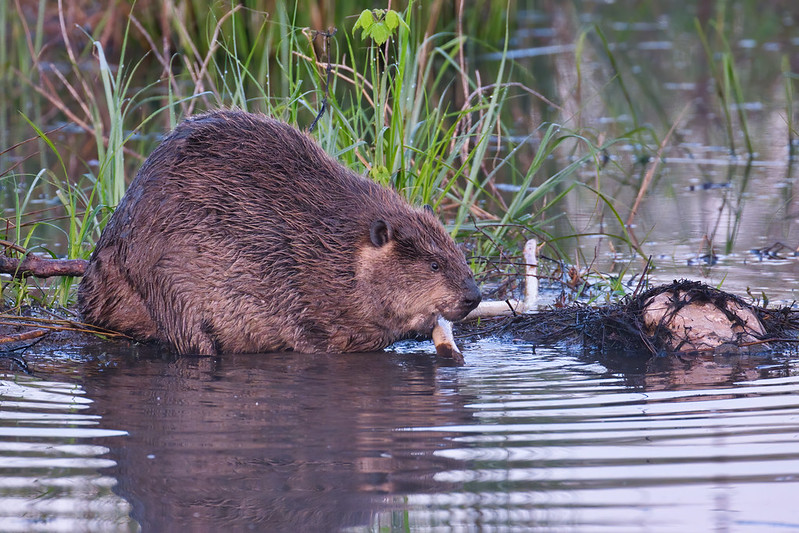In the center of the image, a pudgy beaver with a large arched back is positioned partially in the water on the muddy edge of a small, shallow pond. The beaver has brown fur with a lighter brown underside, beady black eyes, and small ears. It is gnawing on a piece of wood, creating ripples in the clear, wave-less water. Surrounding the beaver, tall green grasses and small plants frame the scene, extending into the blurred background. The overall setting exudes a peaceful, natural environment, emphasizing the beaver’s intricate details and its serene surroundings.